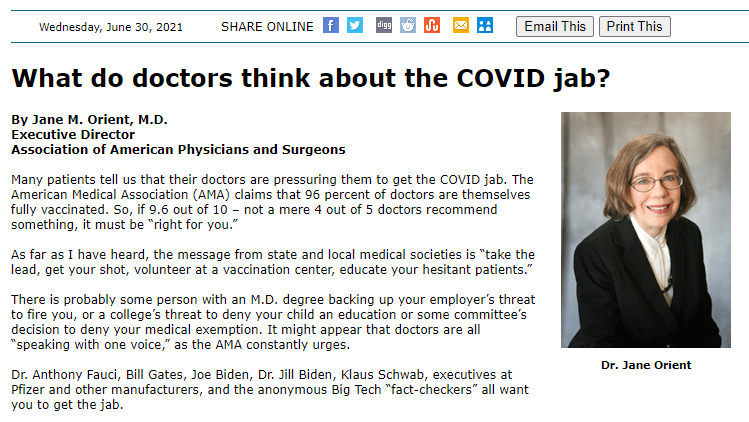**Article Title: "What Do Doctors Think About the COVID Jab?"**

In this detailed image of a news article, prominently titled "What Do Doctors Think About the COVID Jab?", we see various design and information elements. To the right of the article title is a photograph of a woman with short, blondish-brown hair. Her body is angled towards the lower left side of the image, while her head is turned to face the camera. She is wearing glasses, a black coat, and a white shirt. Below the photograph, the caption identifies her as Dr. Jane Orient. 

At the upper left-hand corner of the image, a white bar spans horizontally from left to right displaying the date, "Wednesday, June 30th, 2021." Below the main content of the article, there are several sharing and interaction options inclusive of icons for Facebook, Twitter, Reddit, and email, along with buttons labeled "Email This" and "Print This."